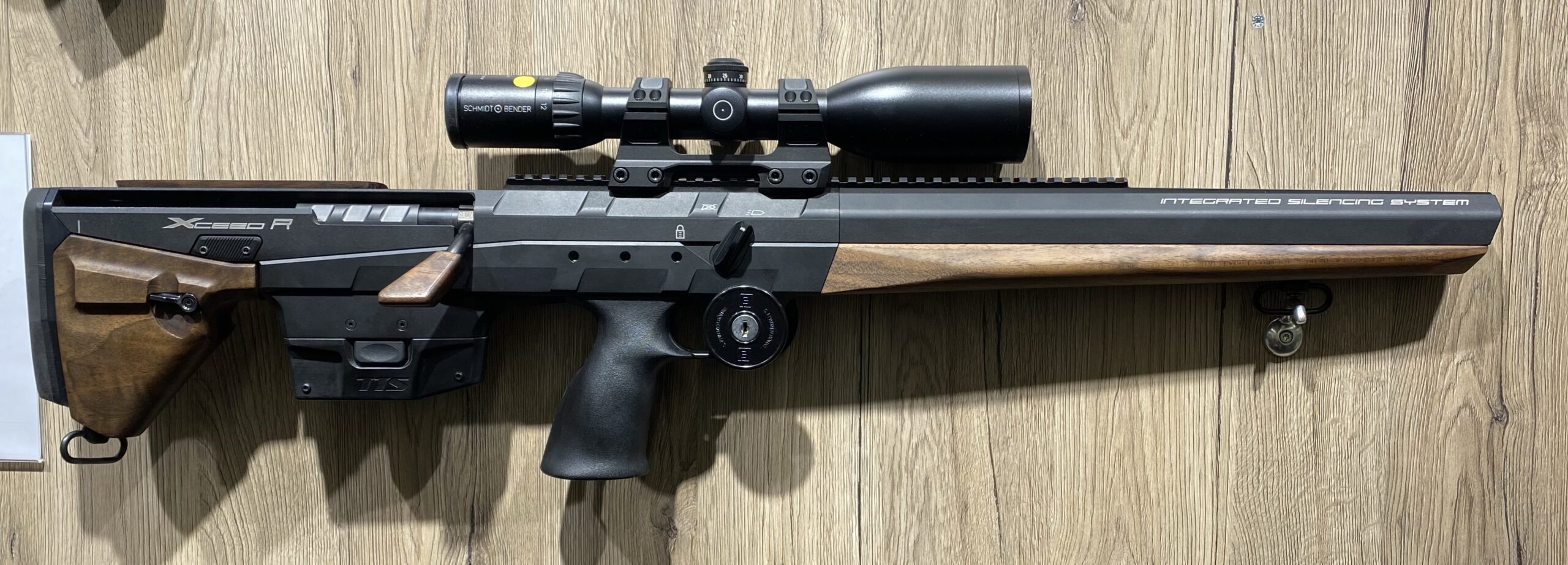This is an up-close, indoor photograph of a short-barreled rifle displayed against a paneled wooden background. The medium-brown wood paneling features black vertical stripes and some bolts or hooks holding the rifle in place. The rifle itself is predominantly black, with intricate wood grain inlays on the stock and underneath the barrel, giving it a distinctive appearance. The barrel is notably short, around 15-17 inches, with the stock nearly matching its length, creating a compact profile. Central to the rifle is a mounted scope inscribed with "Schmidt Bender." Additionally, the rifle features a pistol grip for the trigger, brass attachments for a potential sling, and a couple of dials on its body. The image is taken from a straight-on angle, emphasizing the rifle's detailed craftsmanship and the contrasting textures of metal and wood. The photograph is rectangular, approximately six inches wide and one and a half to two inches high. The inscription "XCDR" is visible on the back of the rifle.